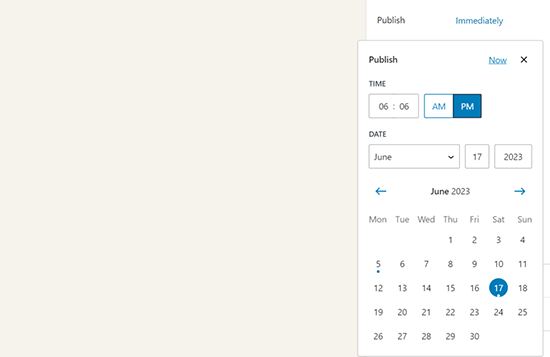A screenshot depicts a user interface for scheduling a publication. The main area occupies the left side, consisting of an empty light gray square. On the right side, a white background presents various scheduling options. At the top, bold text reads "Publish," with the word "immediately" in blue located to its right. Below, a pop-up box features "Publish" on the left and an underlined "now" on the right, accompanied by an X for closing the box.

Further down, a time setting displays "6:06," with selectable options for AM and PM, the latter highlighted in blue with white text. Directly beneath is the date setup, showing "June 17, 2023" in individual boxes, flanked by arrows that allow for date modifications.

A monthly calendar for June 2023 appears at the bottom, enhanced with navigation arrows in blue on either side for switching months. The calendar's text is in black, with a blue circle emphasizing the 17th day.